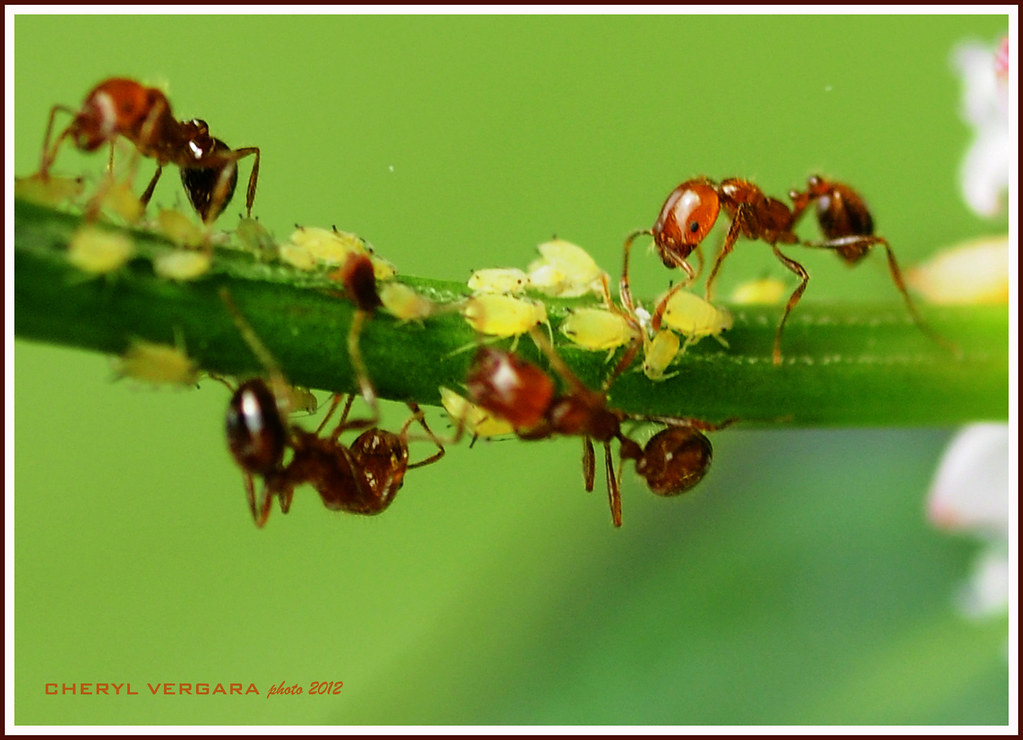This photograph, taken by Cheryl Vergara in December 2020, depicts four red ants in various shades of red and brown, climbing and moving about on a vibrant green plant stem. The ants seem to be interacting or possibly foraging, with two of them positioned on the upper side of the stem and two on the lower side. Small, light green insects, potentially aphids, are also present on the stem, suggesting a complex ecological interaction. The background features a soft green blur due to a strong depth-of-field effect, which emphasizes the detailed foreground activity. The photo also includes a caption in the lower-left corner with red text stating "Cheryl Vergara photo 2020 12," and it is framed in white and black.